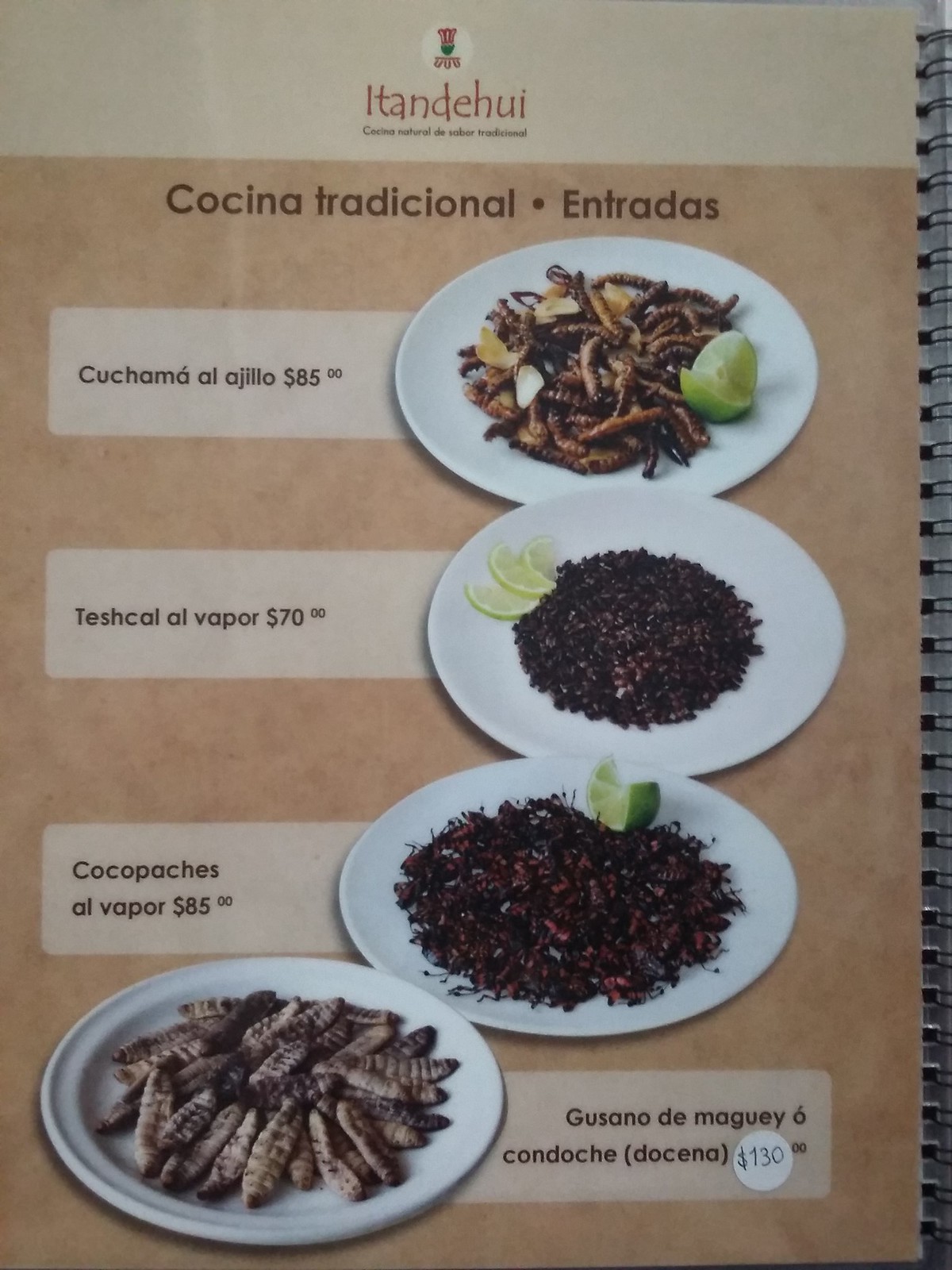The menu, which features a brown background with a faded white border at the top, presents an unappetizing selection of extraordinary dishes. At the top, a red chef figure with a green face is accompanied by a small bubble. Below this figure, in larger lettering, it reads "Ha-Te-Han-De-Hu. Cucata Natural del Sol Tradicional." 

The first dish listed is "Coquina Tradicional Entrenadas." This is followed by "Chumara Alja Agilto," priced at $85, described as a plate of deep-fried mealworms served with a couple of lime slices.

Next, the menu lists "Tejcal del Alevapor," which is a plate of deep-fried fleas, garnished with three small slices of lime positioned in the upper left corner of the plate.

Following that is "Cocopaches al Alevapor," another dish priced at $85. This consists of a plate full of deep-fried cockroaches, again accompanied by lime slices.

Lastly, the menu features "Gusana de Mergo Me Sixto Cocotanche Tequena," priced at $130. This dish is a plate brimming with giant cockroach grubs.

Each dish is described with a white background and black lettering, adding a stark contrast to the overall brown theme of the menu.